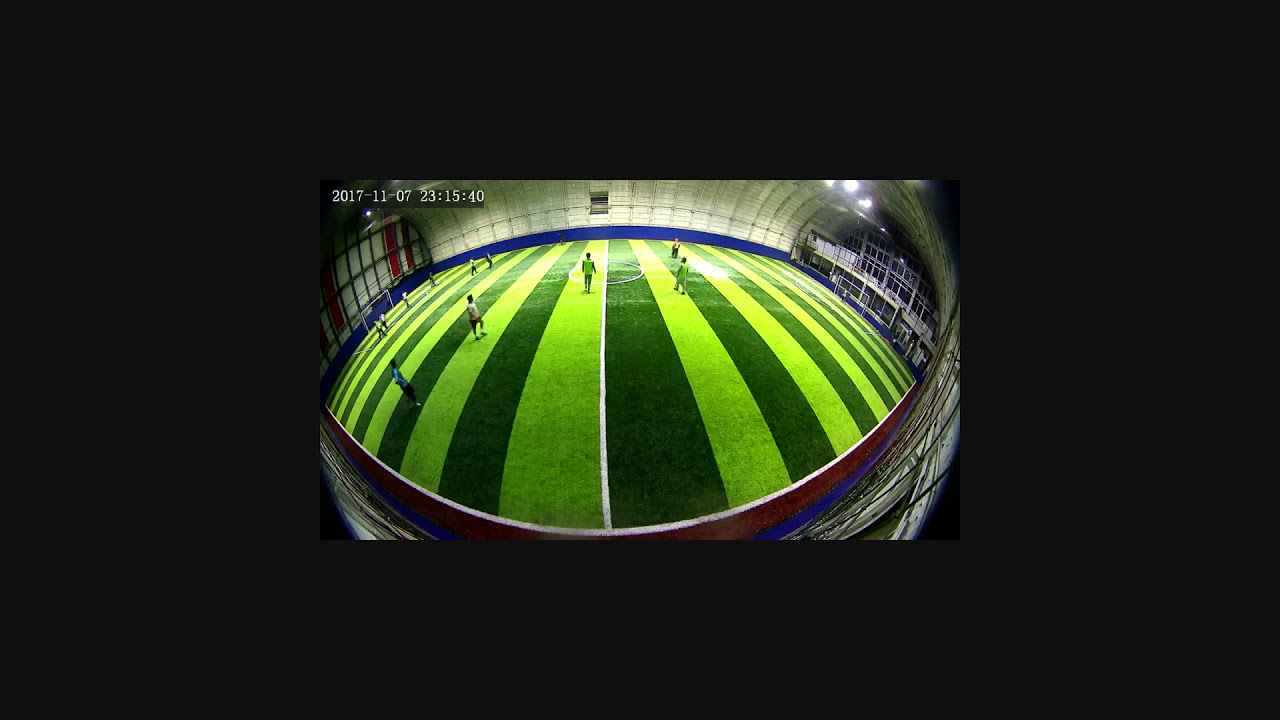The image depicts an overhead view of an indoor soccer field captured with an extreme fisheye lens, creating a distinctive curvy and bent visual effect. The field itself is patterned with alternating light and dark green stripes, reminiscent of a watermelon, and flanked by white goals on either end. The surrounding trim of the field is light blue, leading up to white walls with some red panels interspersed. In the upper left-hand corner, there is a timestamp reading "2017-11-07 23:15:40," indicating the image was taken at a specific date and time. Several people are present on the field, seemingly preparing for a game rather than actively playing, as no one is seen kicking a ball. The facility also features large glass areas, possibly entryways, and some support panels visible around the interior. The image’s main colors are white and green, with an overall impression that the setting may not look entirely real due to the camera's perspective.